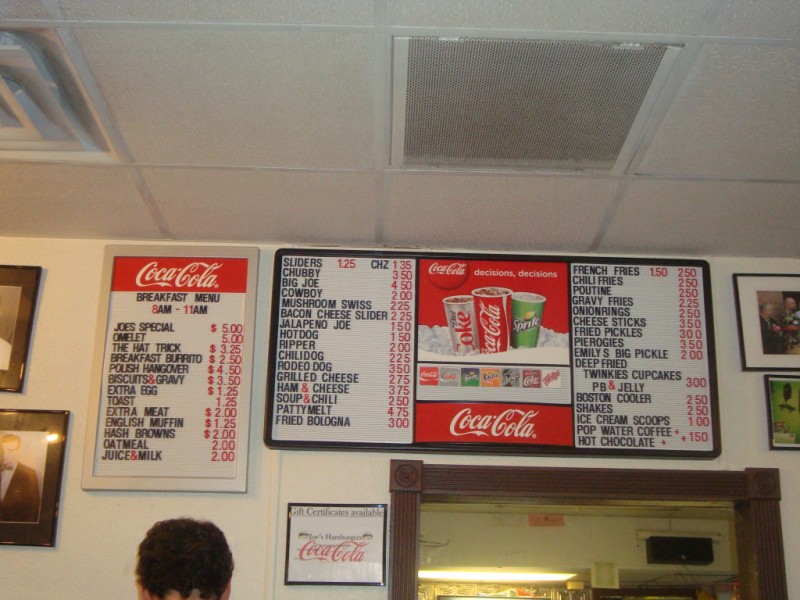In this horizontal image, we see the interior of a quaint, possibly locally-owned fast food restaurant. The establishment features a white drop ceiling with recessed lighting, contributing to the clean and simple ambiance. Dominating the image is the menu board situated above a window that separates the front counter from the kitchen area. The back of a person's head appears in the bottom left corner; they have dark curly hair, but their gender is indiscernible.

The menu board is divided into several sections. To the left is a framed vertical image presenting the breakfast menu, which is available from 8 a.m. to 11 a.m. This section lists items such as Joe's Special Omelette and Hat Trick Breakfast Burritos, with prices shown in red against black text. A label across the top proudly displays the Coca-Cola brand, framed in off-white.

The central menu board spans three panels. The left panel is filled with various food options and their prices: sliders, hamburgers, mushroom Swiss burgers, bacon cheeseburgers, hot dogs, chili dogs, ham and cheese sandwiches, and even fried bologna are listed in vertical rows. The middle panel highlights an assortment of Coca-Cola beverages available in different formats, from cups to cans, featuring options like Coca-Cola and Sprite, with a signature red background and white lettering typical of the brand. The right panel details the side items and miscellaneous offerings: French fries, chili fries, gravy fries, onion rings, cheese sticks, fried pickles, pierogies, "Emily's Big Pickle," Boston Coolers, ice cream scoops, and hot chocolate.

Adding to the nostalgic charm of the restaurant, framed photographs adorn the white wall, likely capturing various moments in the establishment's history. These details collectively paint a vivid picture of a cozy, no-frills eatery serving a diverse menu to its patrons.